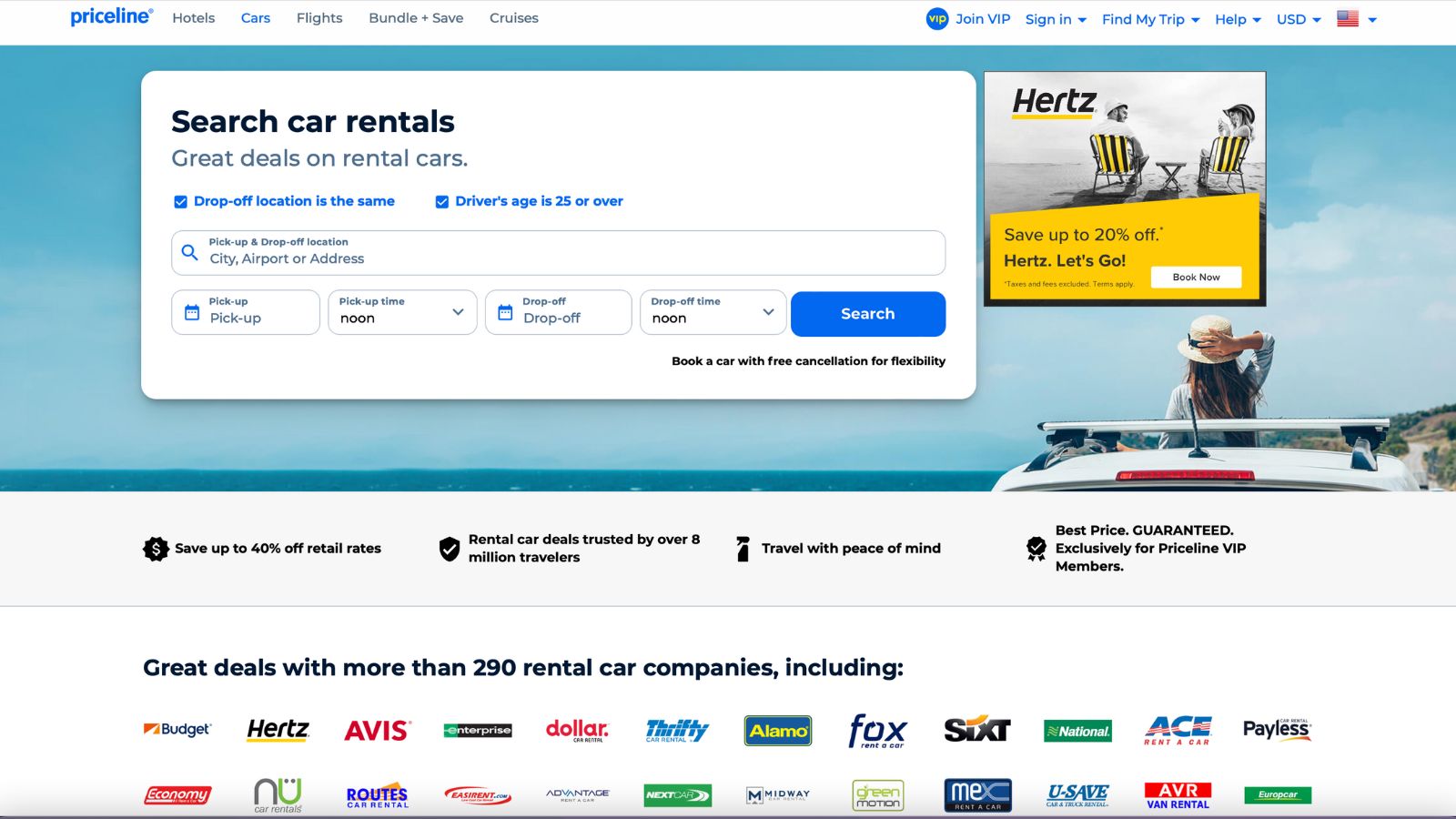**Detailed Caption:**
This image is a screenshot of the Priceline website, prominently displaying the car rental search page. At the very top of the website, there are navigation links allowing users to explore options for Hotels, Cars, Flights, Bundle and Save, or Cruises. The primary section of the screenshot focuses on the car rental search interface. 

At the top of this section, bold black text reads "Search Car Rentals," accompanied by a subtext in gray stating "Great deals on rental cars." Below this, in blue text, the website offers options to check if the drop-off location is the same as the pickup and if the driver's age is 25 or over.

Further down, a search form is visible, beginning with a blank text box for users to enter the pickup and drop-off locations, which can be a city, airport, or address. There are also fields for the pickup date and time, with the time pre-filled as "noon," as well as for the drop-off date and time, also pre-filled as "noon." A prominent blue button labeled "Search" is situated below these fields.

Additional information is provided beneath the search area, stating "Book a car with free cancellation for flexibility," emphasizing the booking's flexibility. At the bottom of the screenshot, there is a reassurance of great deals with over 290 rental car companies, accompanied by a list of icons representing different car rental companies, including Budget, Hertz, Avis, and Alamo.